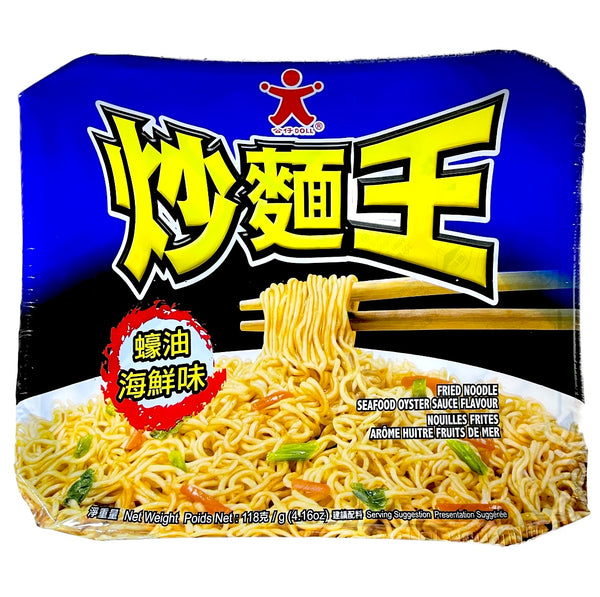The image depicts the front of a rectangular ramen noodle package with truncated corners and slight curvature at the sides. The background transitions from royal blue at the top into a black arc, and then showcases a white bowl filled with beige-ish yellow noodles interspersed with green and orange scraps. Resting above the noodles, tan chopsticks are positioned close together, nearly parallel, with noodles draping from their tips.

At the top, a red, star-shaped figure with white-lined arms and legs is displayed. Beneath this figure is a row of large yellow characters, likely Chinese, which fan outwards and diminish in size towards the center where they overlap the background and part of the chopsticks.

In the middle right section of the image, against the bowl and noodles, is a block of right-aligned text in all caps with white letters bordered in black. The text reads "FRIED NOODLES" at the top, followed by "SEAFOOD OYSTER SAUCE FLAVOUR." Below this in smaller text is an unpronounceable phrase, succeeded by another line suggesting "AROMA NUTRIENTS" or similar wording.

The bottom left features three Chinese characters, followed by "Net Weight Poids Net" in mixed upper and lower case letters. To the right, the package lists "118 G" alongside more Chinese characters. Underneath is the equivalent weight in ounces (4.16 oz) inside parentheses. The minimal, small text at the bottom center-right adds "Serving Suggestion, Preparation Suggestion," hinting at French influence.

Overlaying the left edge of the bowl is a white oval containing yellow Chinese characters with a black background, bordered by a red outline. These graphical and textual elements indicate that the package features an international product, likely Hong Kong style, evidenced by the spelling of "flavour" and the Chinese characters.